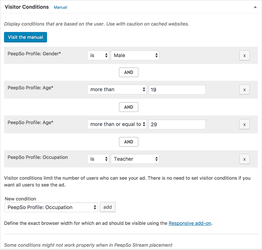The image showcases a web page with a minimalist white background. In the upper left corner, the header features "Visitor Conditions" in bold gray text. Adjacent to this, the word "Manual" appears in bright blue, drawing attention. Below this header, a line of gray text provides instructions: "Display conditions that are based on the user. Use with caution on cached websites."

Directly beneath these instructions, there's a prominent bright blue button labeled "Visit the manual" in white text, inviting interaction.

A horizontal gray ribbon spans across the page, containing the text "People Profile Gender" in gray. Under this section, there are two boxes aligned side-by-side: the first box has a drop-down menu labeled "Is," and the second box has another drop-down menu marked "Male."

Further down, a white space adorned with the word "And" encased in a gray border divides the content. Below this space, another light gray ribbon labeled "People Profile Age" appears. This section includes two white boxes: the first box reads "More than," while the second box specifies "19."

Repeating the pattern, another white space with the word "And" in a gray-bordered box is present below. Following this is an additional gray ribbon labeled "People Profile Age." In this section, the first white box text reads "More than or equal to," accompanied by a drop-down menu, and the second box states "29."

This webpage layout appears to be specifically designed to refine and display user conditions based on gender and age criteria.